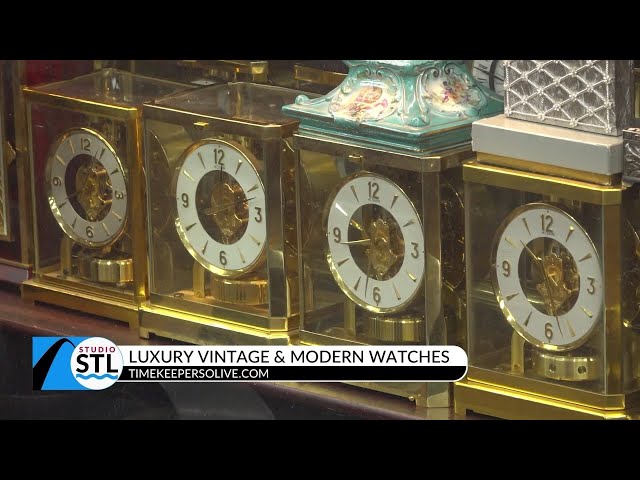The image showcases a display of vintage and modern luxury clocks. Prominently featured are four elegant, rectangular prismic analog clocks set in gold-rimmed glass cases, each with intricate exposed gears visible through cutouts in their white clock faces. The clocks are neatly arranged in a row, each with gold numbers and set on square metal bases. On top of the two rightmost clocks are additional rectangular-shaped objects, possibly vases or lamps, with one being green with white designs and the other gray or silver. The photo includes black horizontal bars at the top and bottom, with text overlaid on the lower half, reading "Studio STL Luxury Vintage and Modern Watches," followed by the website "TimekeeperSolive.com." The text suggests a connection to St. Louis, potentially indicated by a graphic resembling the Gateway Arch of the city.